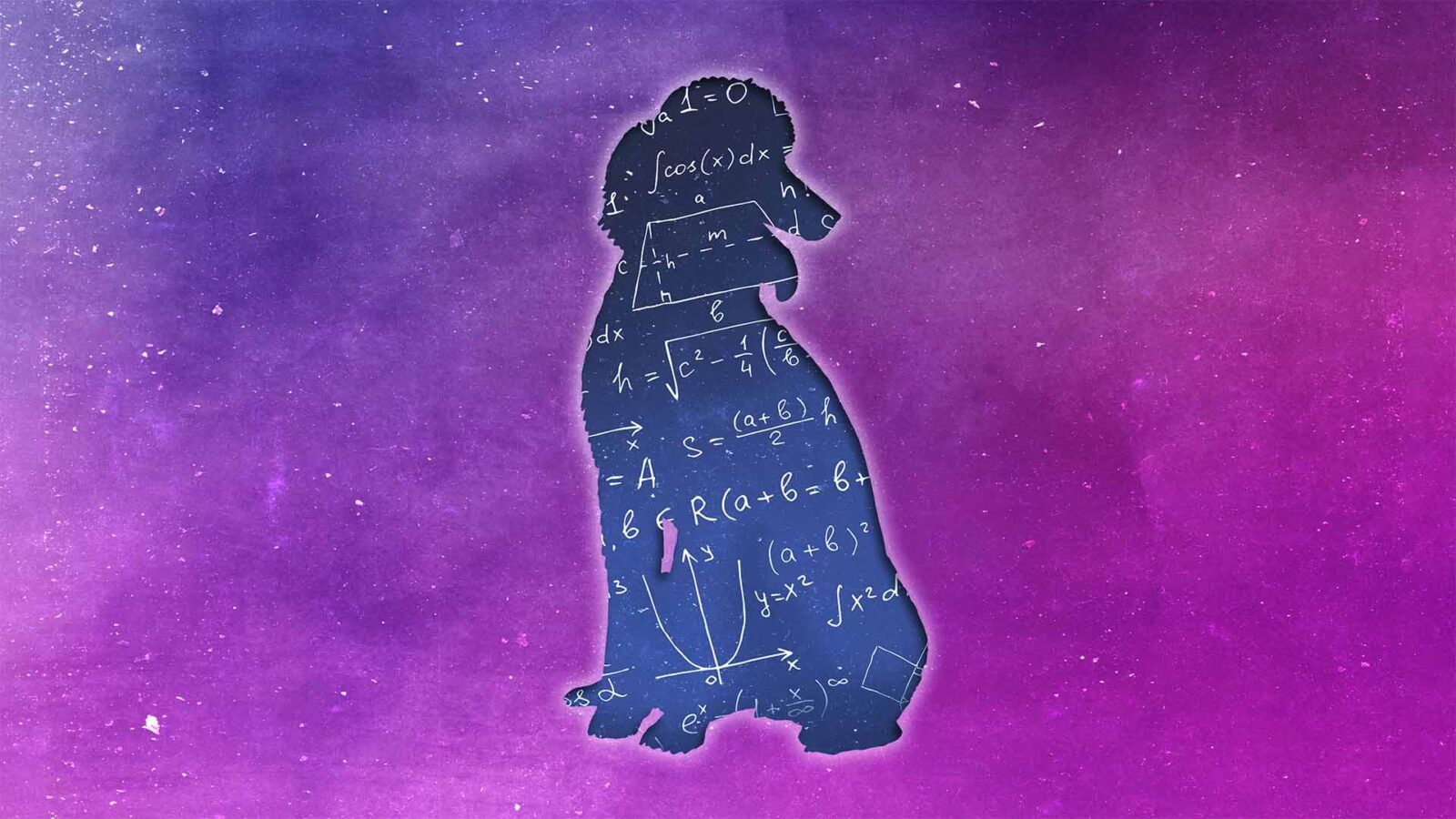The image portrays a large rectangular space with a bluish-purple background that resembles an exaggerated night sky filled with numerous stars. At the center of this artistic portrayal is the cutout shape of a full-size poodle, sitting down and looking to its left (our right). The poodle’s shape is filled with a blackboard-like surface covered in white mathematical equations, including various geometric and calculus formulas such as "S = A + 6 over 2 H" and "1 over 1 H minus negative M." Highlighting its detailed nature, the poodle cutout also features a representation of a tongue hanging out, contributing to its lifelike appearance amidst the abstract cosmic setting.